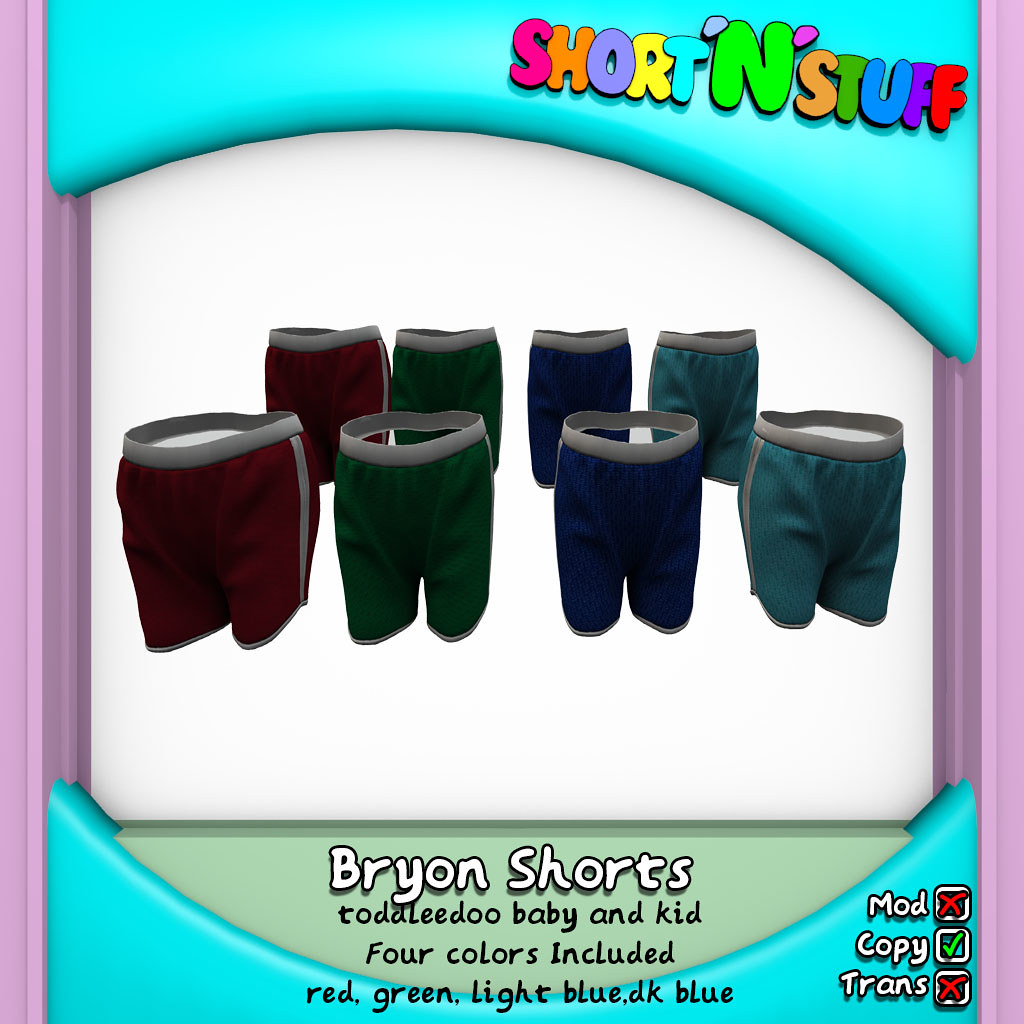The advertisement features a colorful display for the product "Bryon Shorts," aimed at children. The image's background transitions from purple on the left and right sides to a turquoise blend at the top. Dominating the upper-right corner is a slanted, curved banner in a teal color, displaying the multicolored, bubbly text "SHORT'N STUFF." The letters are arrayed in a vibrant rainbow of colors, including shades of pink, orange, purple, yellow, turquoise, green, dark green, dark blue, dark purple, and red.

At the center, set against a stark white background, there are two neat rows of shorts, each row presenting four pairs. The shorts, available in red, green, light blue, and dark blue, appear in two pairs of each color. Notably, the shorts in the front row are slightly open in the back, revealing details behind them. Below this array, text spells out "Bryon Shorts" and details their product variants: Toto, Lido, Baby, and Kid, available in four distinctly mentioned colors.

In the bottom part of the image, there are three checkboxes in the lower right-hand corner, each labeled Mod, Copy, and Trans. The box labeled Mod and the box labeled Trans are marked with red Xs, while the box labeled Copy has a green check mark.